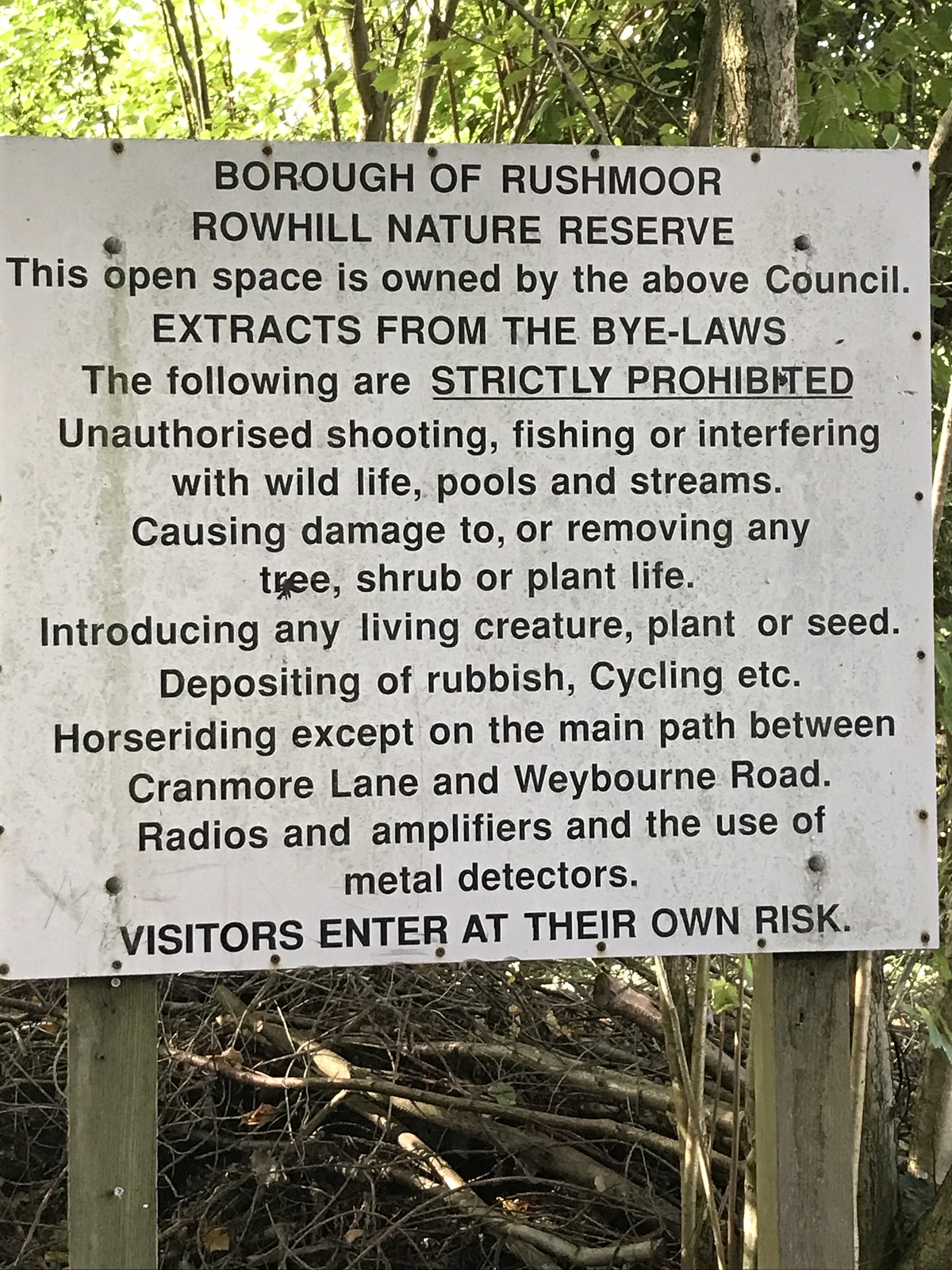This image depicts a weathered white sign with black text, fastened by rusty screws to two wooden posts that appear greenish-brown, signifying mold or weathering. The sign, located in a wooded area with light filtering through leaves and branches, bears the following text in capital letters at the top: "Borough of Rushmore Roehill Nature Reserve." Below this, in mixed capitalization, it states, "This open space is owned by the above council. Extracts from the bylaws." Further down, sections in varying capitalizations and underlining read: "The following are strictly prohibited: unauthorized shooting, fishing, or interfering with wildlife, pools, and streams; causing damage to or removing any tree, shrub, or plant life; introducing any living creature, plant, or seed; depositing of rubbish, cycling, etc.; horse riding except on the main path between Cranmore Lane and Wayburn Road; radios and amplifiers; and the use of metal detectors." At the very bottom, the sign concludes with an all-capital warning: "Visitors enter at their own risk." The base of the posts rests among dead branches and sticks on the ground.